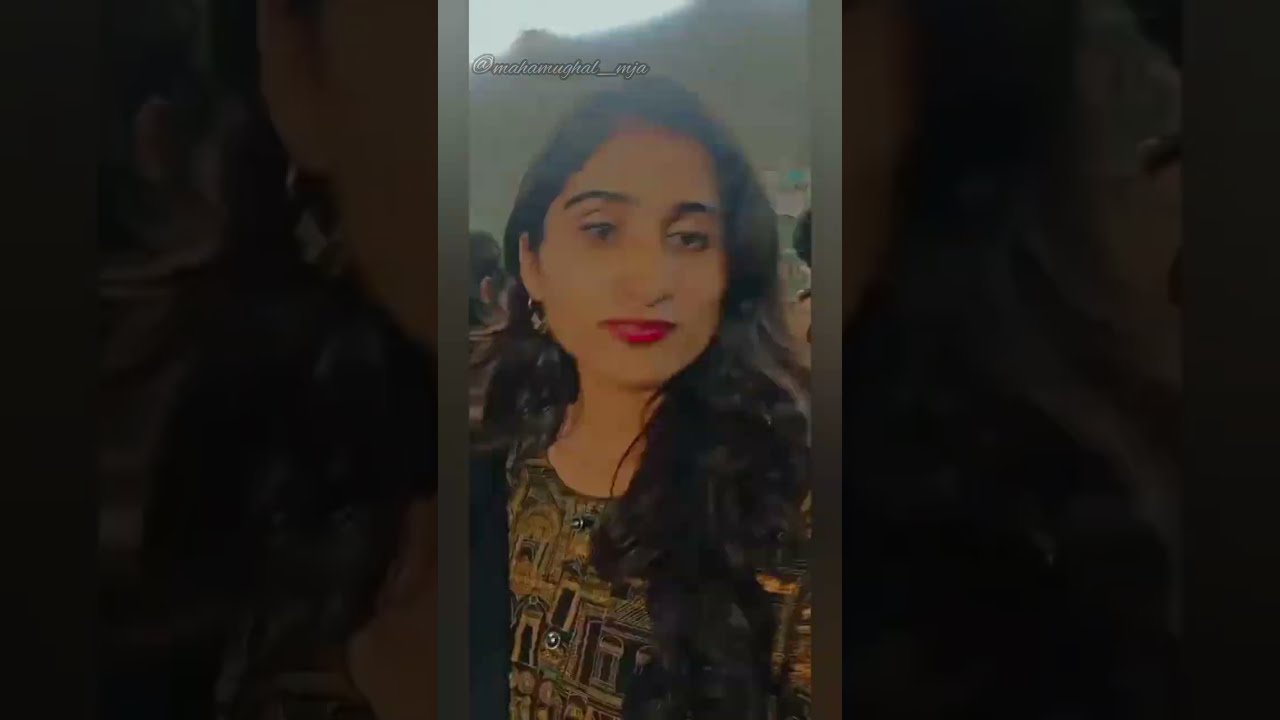The image is a somewhat blurry and dark color photograph taken in portrait mode, capturing a woman taking a selfie. Her social media handle, @mahamughal_mja, is prominently displayed at the top. She has long, wavy, black hair, adorned with an earring visible on the right side. She wears heavy makeup, including dark eyeshadow, dark eyebrows, and striking red lipstick. Her outfit consists of a black and dark green blouse with a distinct pattern, featuring tight squares that create an almost architectural effect. The blouse has a few buttons near the collar, and she appears to be wearing either an armband or a black sweater over it. The photograph's background is somewhat indistinct, revealing the heads of several people behind and around her, possibly in a room with a grayish wall or ceiling. Additionally, the edges of the photo are darkened with enlarged and grayed-out details from the central image, creating a thick border on both the left and right sides.